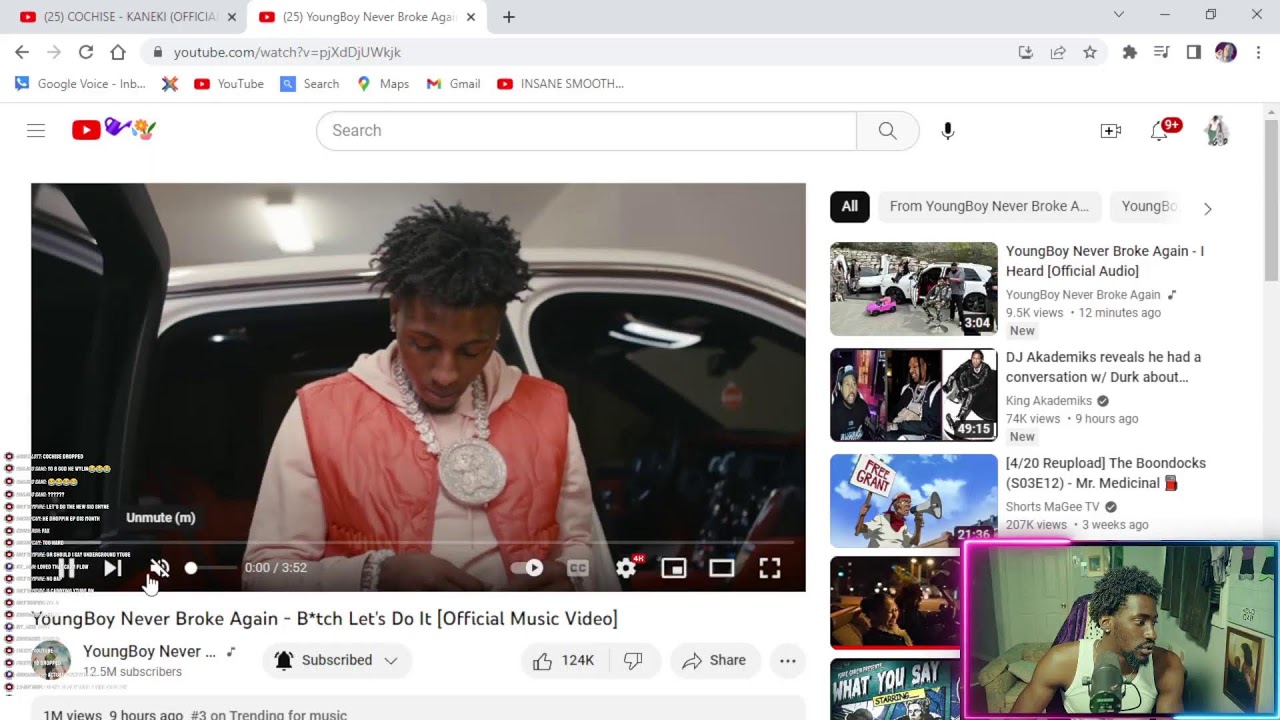The image showcases a popular YouTube channel open in a Google Chrome window. The defining features of Google Chrome, including its distinct interface, are easily recognizable. The user, an African-American male, appears in the bottom right corner of the screen, seemingly engaged but looking off to the side. Multiple tabs are open along the top left of the browser, with the current tab focusing on a paused music video. Another music video tab is also visible. The video's audio is muted. Surrounding the main content, YouTube suggests various recommended videos aligned with the viewer's musical interests. Additionally, the top of the screen features a notification bell icon with a red alert, indicating pending notifications.